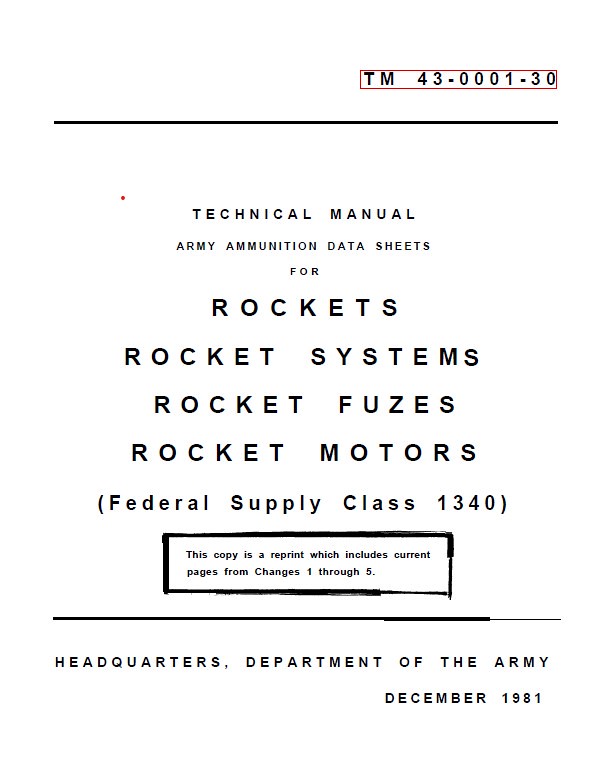The photograph displays a white background with centered black text across it. In the upper right corner, it reads "TM43-0001-30," enclosed in a red frame. Directly below, there is a narrow black line running the width of the page. Centered beneath this line, the text reads: "Technical Manual," followed by "Army Ammunition Data Sheets for Rockets, Rocket Systems, Rocket Fuses, Rocket Motors." Enclosed in parentheses is "Federal Supply Class 1340." Below this, there is a hand-drawn black box containing the text: "This copy is a reprint which includes current pages from changes 1 through 5." Another black line runs beneath this box, and at the bottom of the page, it states: "Headquarters, Department of the Army, December 1981."